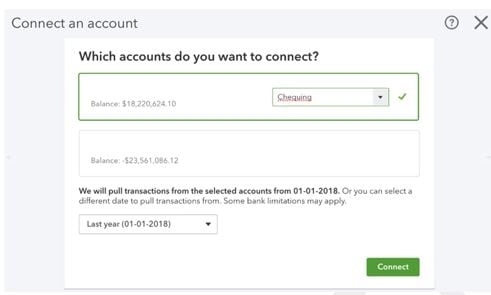In the image, we see a screenshot of a financial management interface. The interface consists of a light gray rectangular background. In the upper left corner, the text "Connect an Account" is displayed in gray font. On the upper right corner, there is a small gray circle with a question mark inside it, and immediately to its right, a gray 'X'.

Centered below that, in bold black text, is the question, "Which accounts do you want to connect?" Beneath this question, there's a box outlined in green, which contains the text "Balance: $18,220,624." To the right of this green-bordered box, there is a dropdown menu labeled "Checking," accompanied by a green check mark.

Further down, another statement in bold black text reads, "We will pull transactions from the selected accounts from 1-1-2018, or you can select a different date to pull transactions from. Some bank limitations may apply."

In the lower right corner, there is a prominent green action button labeled "Connect."